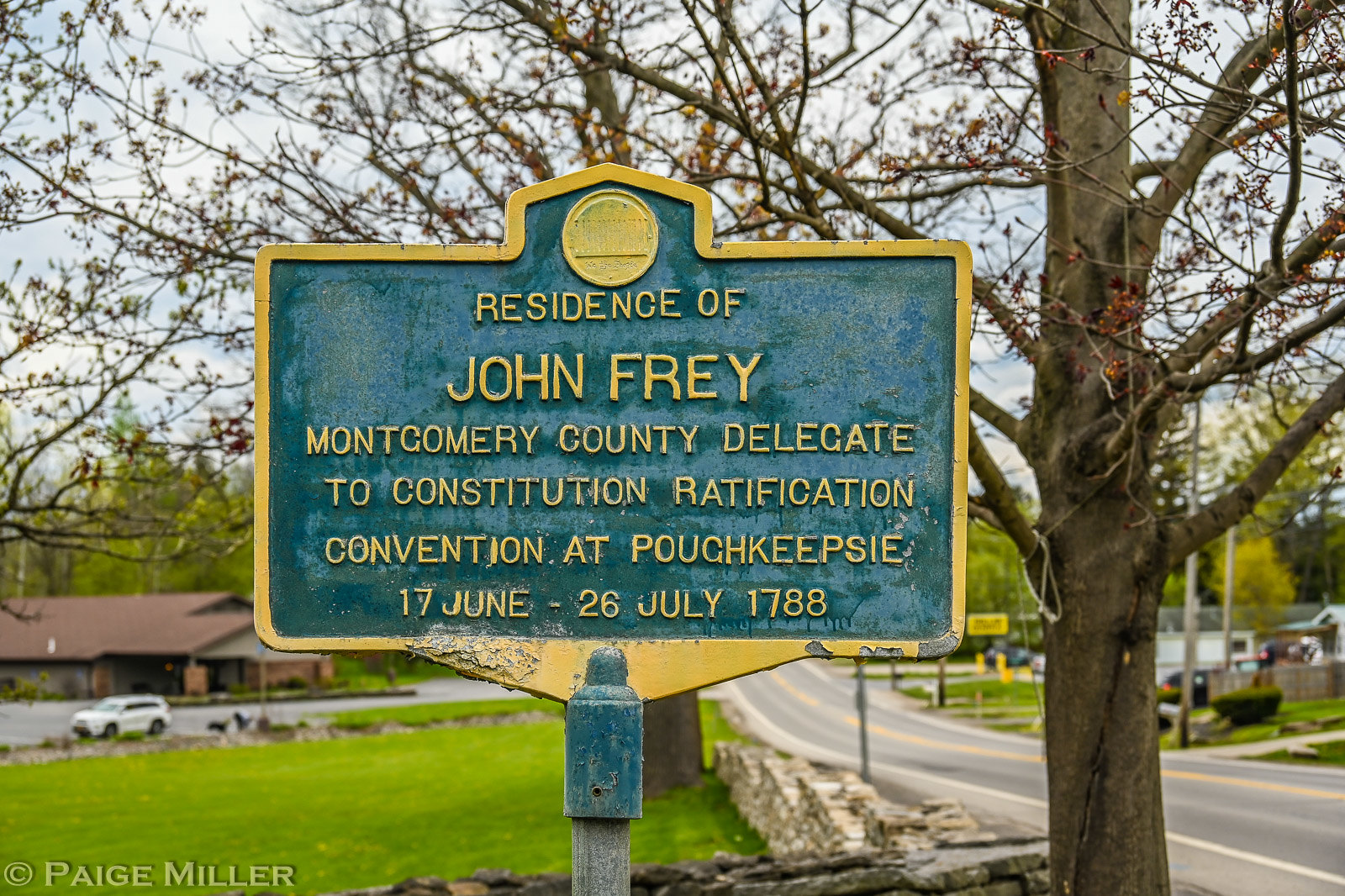This image, copyrighted by Paige Miller, showcases a historical metal sign with a distinctive blue-green background and gold lettering, detailing the residence of John Frey, Montgomery County Delegate to the Constitution Ratification Convention at Poughkeepsie from June 17 to July 26, 1788. The sign, mounted on a metal pole, features a rectangular shape with rounded edges, and its golden details are weathered and chipping. It is positioned near a stone wall, with a large, leafless tree to its right. The setting includes a scenic view of a green lawn extending to a road lined with white and yellow markings. In the background, one can spot a house with a parked white car, possibly a store to the right, and stacked wood, all contributing to the quaint, historical atmosphere of this residential area. The image also has a watermark in the bottom left corner indicating Paige Miller's copyright.